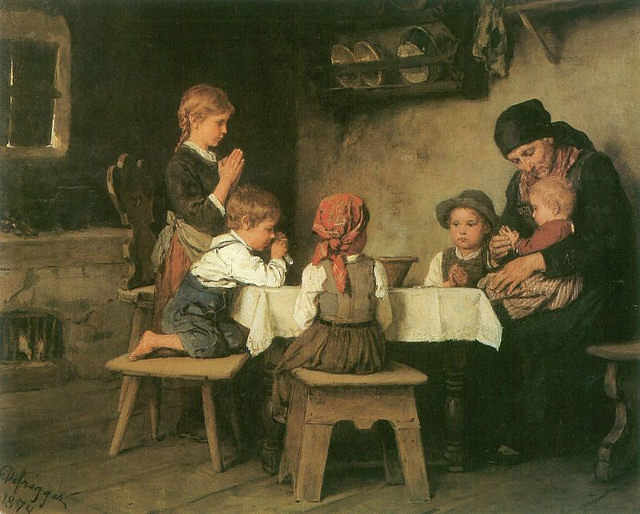This detailed image depicts an 1800s family gathered around a modest wooden table adorned with a white tablecloth that has delicate lace trim at the bottom. At the center of the image, the mother, dressed in a black dress and headband, tenderly cradles a young child, who appears to be around a year to a year-and-a-half old. Seated beside her is another child, approximately four or five years old, and an additional child possibly around the age of six. The eldest child, a girl about 11 years old, stands with her hands clasped together in prayer, suggesting that the family is engaged in a moment of blessing before a meal. The table, with black legs, features a bowl at its center, indicative of a humble setting.

Surrounding the family, the background reveals more of their simple home. To the left, a stone fireplace can be seen, although it intriguingly houses a cage with chicken instead of a fire. Above the table, there's a shelf lined with dishes. The wooden stools or chairs add to the rustic charm of the scene. Light brown wooden flooring and a window in the background further enhance the warm, homely atmosphere.

The image also bears an artist's signature at the bottom left, indicating the year 1890, and it showcases a palette of colors including light brown, orange, red, pink, maroon, black, white, and various shades of gray, which give the artwork a hand-painted feel. There is no father present in this intimate family moment, perhaps suggesting he is out working. The overall composition is rich with historical and familial detail, capturing a serene and poignant snapshot of 19th-century life.